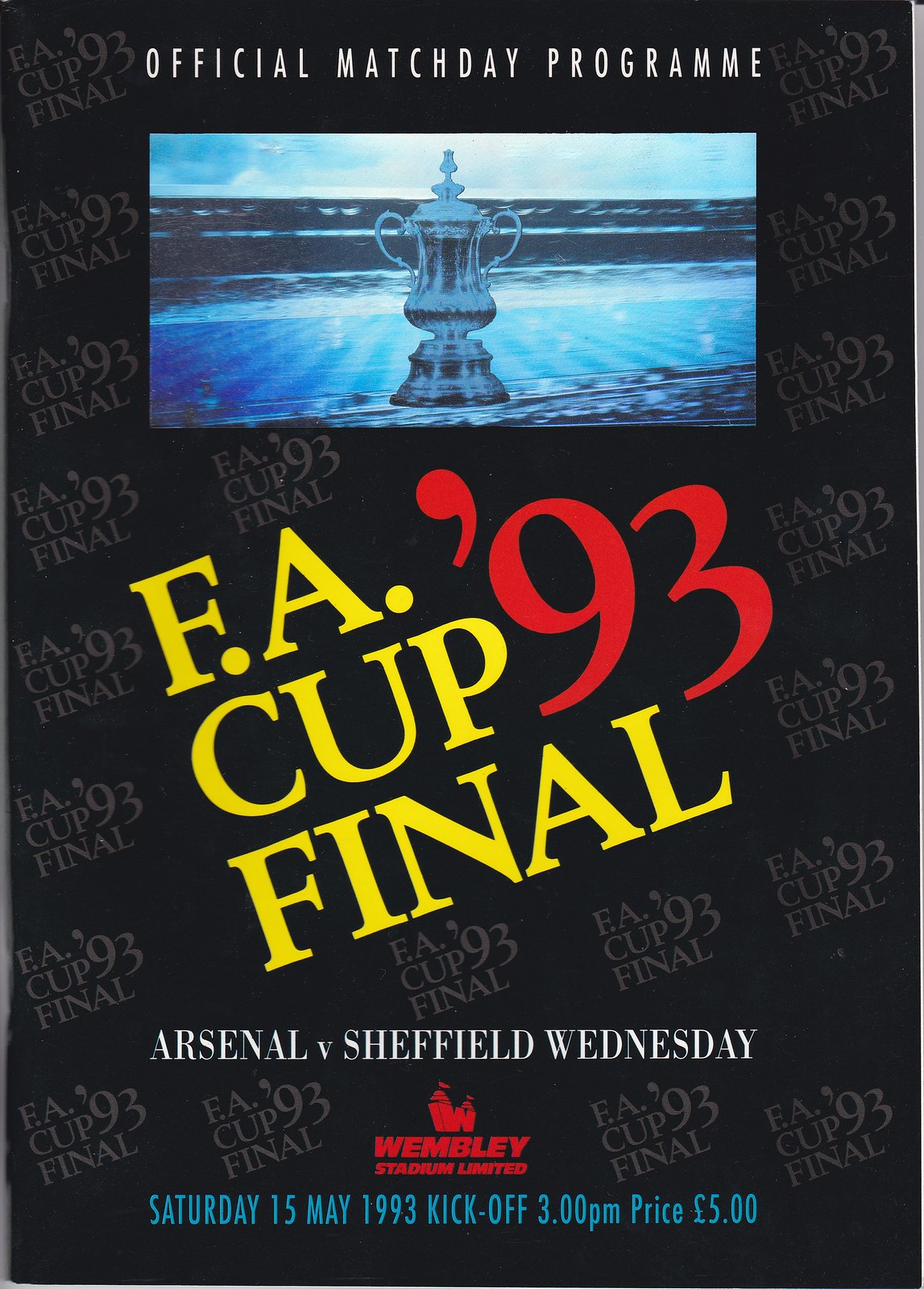Official match day program for the FA Cup Final 1993 between Arsenal and Sheffield Wednesday, held at Wembley Stadium Limited on Saturday, May 15th, with a kickoff at 3 p.m., priced at five pounds. The program features a black background adorned with multiple "FA Cup Final 93" imprints in lighter, grayish text. Prominently displayed in the center is a trophy, presumably the FA Cup, set against a detailed backdrop. At the top of the program, "FA Cup Final" is presented in yellow text, with "'93" in red, slightly tilted. Below that, in white text, it states "Arsenal vs. Sheffield Wednesday." Near the bottom, a red emblem of Wembley Stadium Limited is visible, with additional details in blue text specifying the date, time, and price.